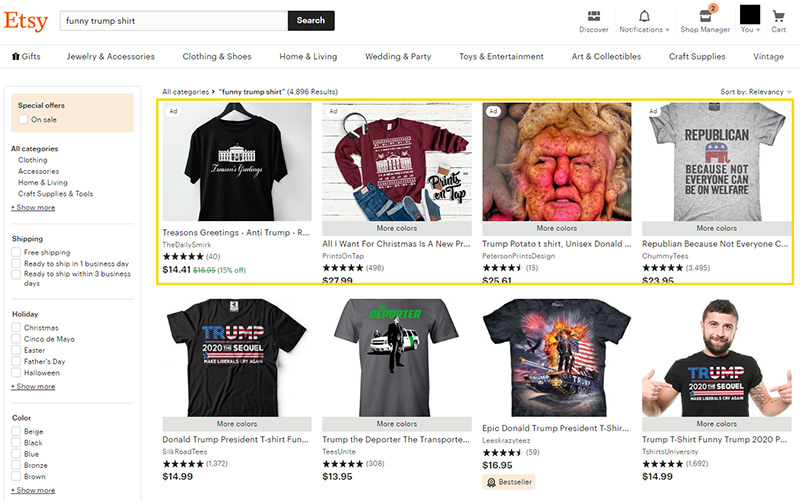This image is a screenshot captured from a webpage on the Etsy website. In the top left-hand corner, the company's name, "Etsy," is prominently displayed in a distinct dark orange-colored font. Adjacent to the logo is a search bar containing the text "Funny Trump Shirt." Spanning the majority of the image are two rows of t-shirts, each row displaying four different shirts. All the shirts pertain to Donald Trump and the Republican Party, featuring various designs and slogans related to these themes.

On the left side of the image, there is a filtering panel offering different categories, shipping options, and color selections. This panel enables users to refine their search results based on their preferences. In the top right-hand corner of the screenshot, a series of icons are visible: a cart button for viewing items in the cart, a profile button for user account settings, a notification button, and a shop manager button. The shop manager button is marked with the number two, indicating two pending notifications.

The entire webpage has a clean, white background, providing a simple and uncluttered interface for browsing products on Etsy.